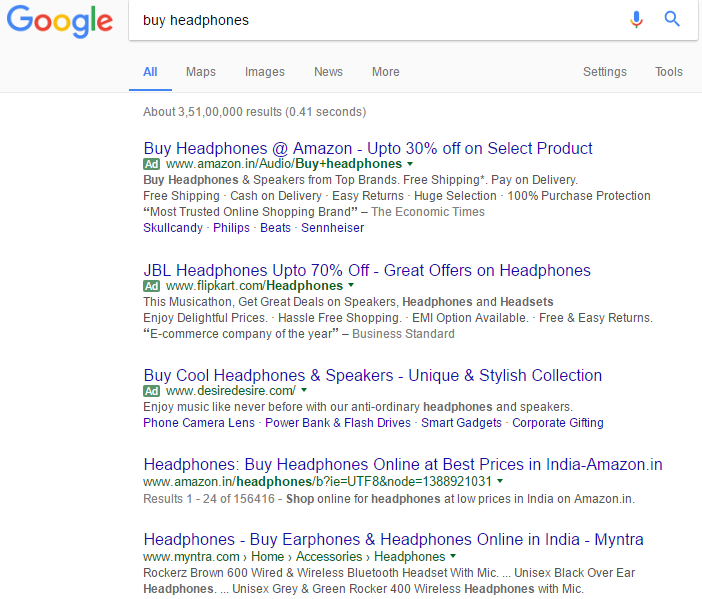This image features a Google search results page displayed on a computer screen. In the top left corner, the iconic multicolored Google logo is clearly visible. The search query entered into the search bar reads "buy headphones," and to the right of the search field, the microphone icon and the magnifying glass icon for searching are displayed. Below the search bar, menu options for refining the search results include: All, Maps, Images, News, More, Settings, and Tools. The results indicate about 3,510,000 entries, although the exact number of digits may be incorrect.

The first search result is an advertisement from Amazon, offering headphones with up to 30% off on select products. The ad includes links to popular brands such as Skullcandy, Philips, Beats, and Sennheiser. The second result highlights JBL headphones with up to 70% off, mentioning great offers on their products. The third result points to a unique and stylish collection of headphones and speakers available on www.ingreen.desiredesire.com, with additional information about other products such as phone camera lenses, power banks, flash drives, smart gadgets, and corporate gifting options.

Further down, another result directs users to buy headphones online at the best prices in India via Amazon, with the website details presented in green text. Finally, the last result mentions buying earphones and headphones online in India through Myntra, also featuring the website details in green and providing information about the available products.